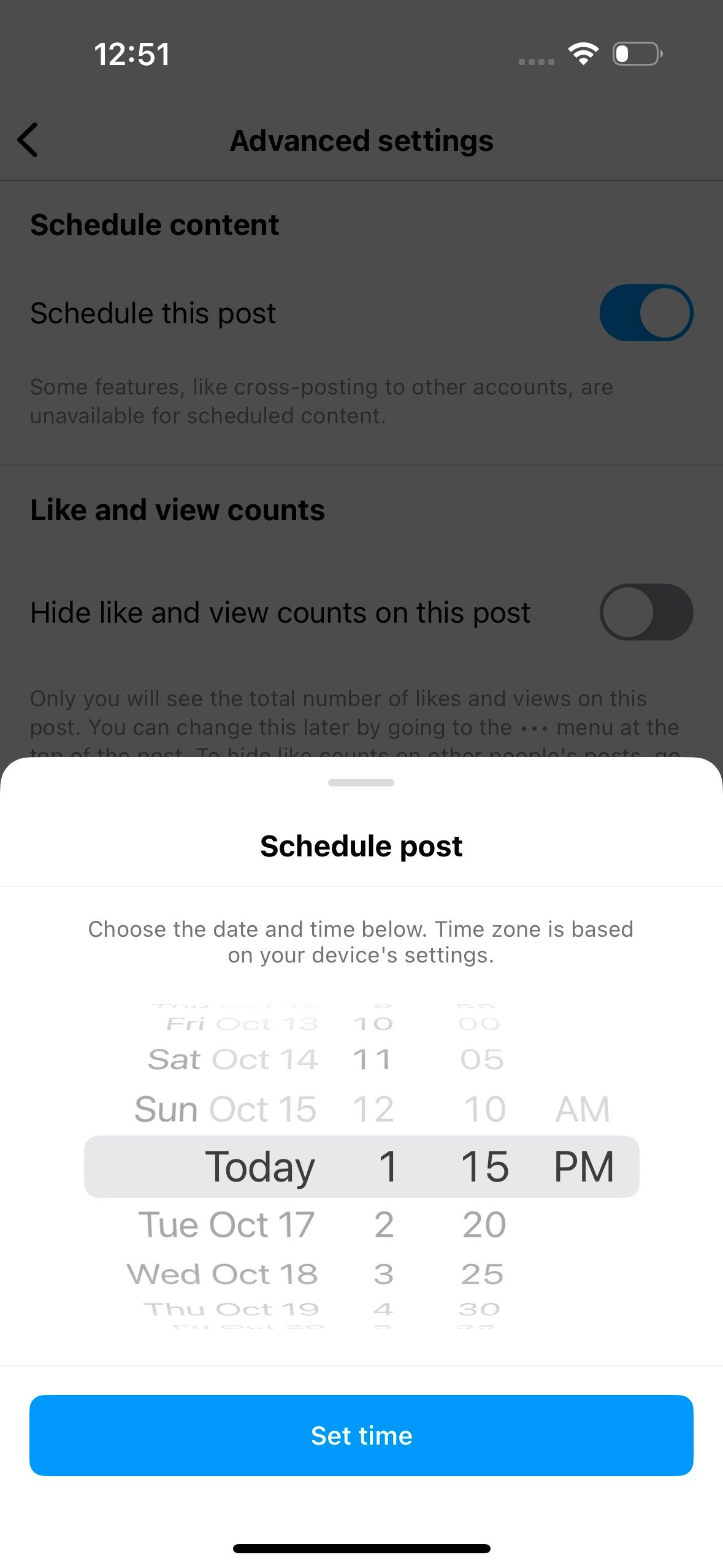This image is a screenshot from a smartphone displaying a scheduling interface for a post. The top half of the screen is overlaid with a gray shadow, while the bottom half features a white background housing a pop-up window.

In the top left corner, the current time is displayed. The top right corner contains a quarter-full battery icon, a Wi-Fi symbol, and four gray dots. Below the time, a black greater-than symbol points to the right. Centered and bolded in black text is "Advanced Settings," with "Scheduled Content" to its left and slightly lower. Directly below, there's a toggle switch for "Schedule this post," which is turned on and colored blue.

Further down, two small-print lines precede another bolded section titled "Like and View Counts," under which there's an option to "Hide like and view counts on this post," currently toggled off. Following this are two more lines before the pop-up portion starts.

The pop-up begins with a small, centered gray line at the top. Below this, "Schedule Post" is bolded, followed by the instruction "Choose the date and time below." It notes that the time zone is based on the device settings. A date and time selector resembling a Rolodex is displayed, starting with "Saturday, October 14th, 11:05 AM."

Next, "Sunday, October 15th, 12:10 AM" is shown in plain black text on a white background. The currently selected time, "Today, 1:15 PM," is highlighted within a gray rectangle with bolder black text. Following entries include "Tuesday, October 17th, 2:20 PM," "Wednesday, October 18th, 3:25 PM," and "Thursday, October 19th, 4:30 PM," gradually fading towards the bottom.

Beneath this list is a large blue button labeled "Set Time" in white text. Finally, there's a black bar centered horizontally about an inch from the bottom, extending slightly left and right.